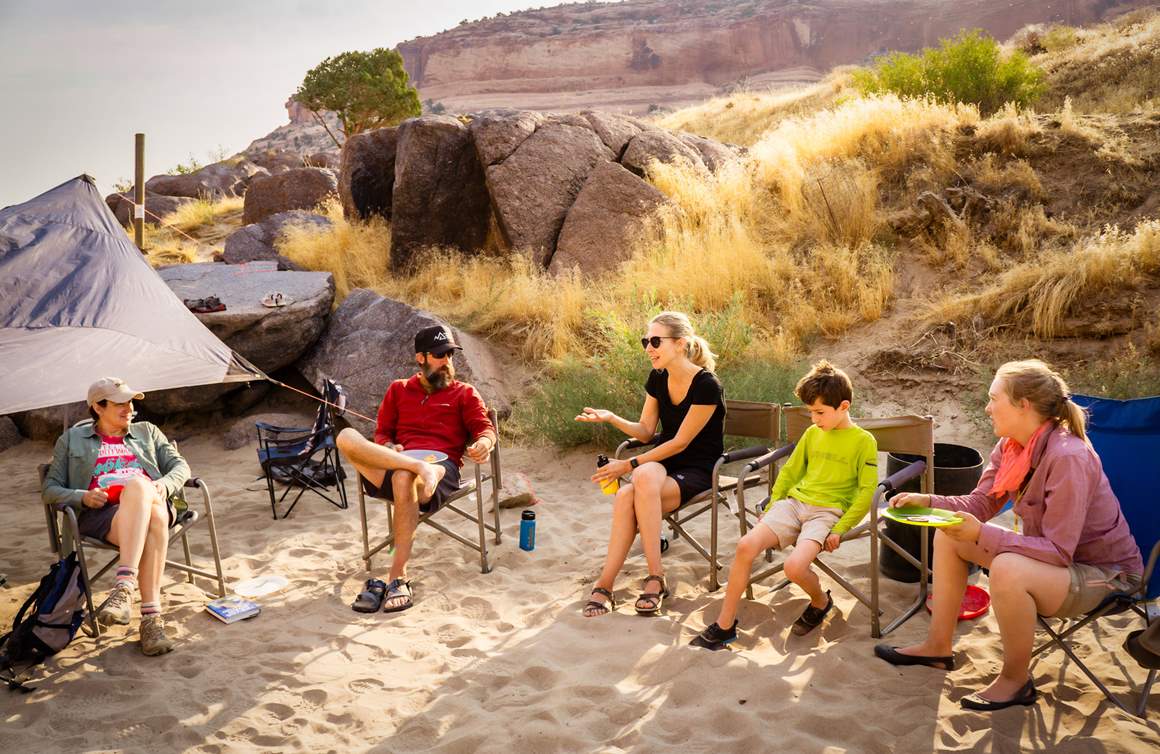This photograph captures a serene family gathering at the beach, where five individuals sit in a semicircle of folding chairs positioned on the sandy ground. Starting from the left, a woman in her thirties, wearing a tan ball cap and sunglasses, sits with her legs crossed. Next to her is a man—possibly her husband or father—wearing a black ball cap and sunglasses, with a large beard. To his right sits a woman in her thirties also donning sunglasses; she gestures as she talks, holding a water bottle in her left hand. Further along is a young boy, approximately ten years old, dressed in a lime green long-sleeved shirt and sandals. Completing the semicircle is a woman in her fifties, who sits turned towards the group, holding a plate, indicating a recent meal. 

A taut tarp, providing shelter and shade, is visible to the left of the group. The background features a large rock outcrop rising from the tall, yellow grass, with one or two green bushes scattered nearby. In the distant backdrop, a vast rock ledge or ridge can be seen, adding depth to the scene. Despite being in the remote sandy area, the family's peaceful demeanor stands out, accentuated by the natural beauty surrounding them.